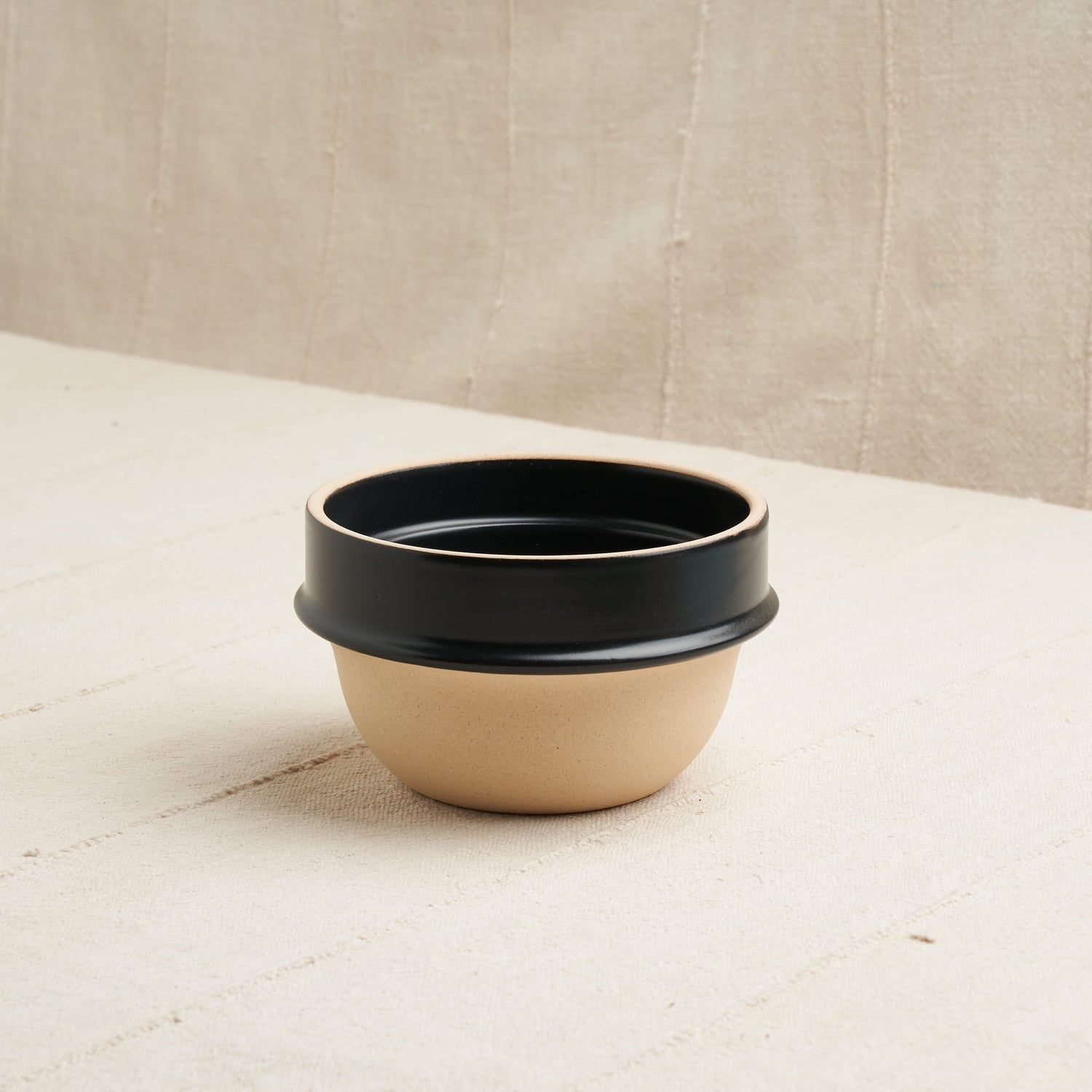This square photograph captures a minimalistic scene with a white surface, which could be a table or a deck, at the bottom. Centrally placed on this surface is a light brown or tan bowl. Resting atop the bowl is a small, cylindrical, black object with an open top. The background features a white wall adorned with vertical lines that resemble a wooden fence or paneling, contributing to the overall simplicity and structure of the image. The bowl and the cylindrical object create a unique juxtaposition against the clean, lined backdrop, highlighting the elegant minimalism of the composition.